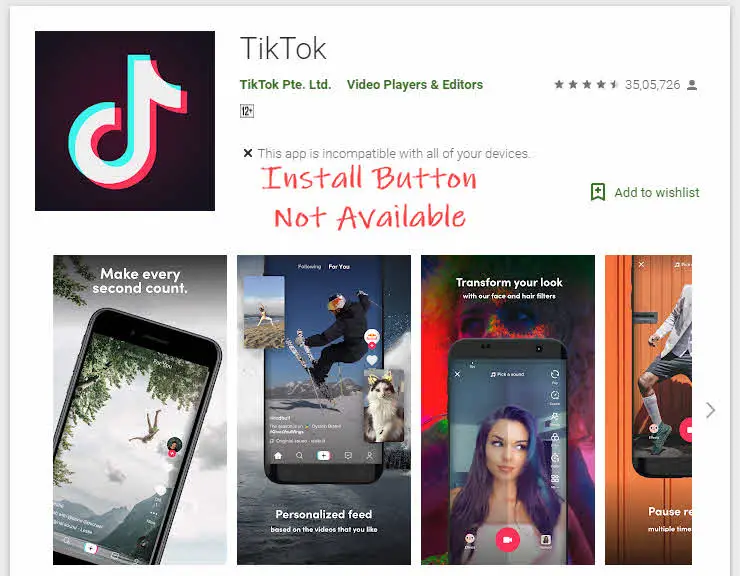This image depicts the TikTok app listing on a digital store interface. On the left side of the image, there is a prominent black square. Overlaid within this square is the iconic TikTok symbol, resembling a stylized musical note with a seahorse-like curvature, set against a gradient background of blue and red hues. Below the logo, it reads "TikTok PT-LTD," accompanied by the category "Video Players & Editors."

Rating information is displayed as a series of stars, enumerated as 1, 2, 3, 4, with a cumulative rating from millions of users, exactly "35,726,000,000." The review section features an avatar symbolizing user feedback.

A message indicates, "This app is incompatible with all your devices," and the usual "Install" button is conspicuously absent, prompting the viewer with an option to "Add to Wish List" instead.

Adjacent to this message, there's a visual placeholder where the "Install" button would typically appear. Below, a highlighted slogan reads, "Make Every Second Count," which showcases a smartphone actively recording a video as part of the promotional content.

Further down, additional promotional snippets describe features like "Personalize Your Feed," highlighting that the app customizes video recommendations based on user preferences. Another feature touts the ability to "Transform Your Look with Our Face and Hair Filters," augmented by an arrow indicating more options and functionalities.

Overall, the image serves as a comprehensive advertisement for TikTok, emphasizing its primary functions, personalization options, and current device compatibility issues for the user viewing the listing.